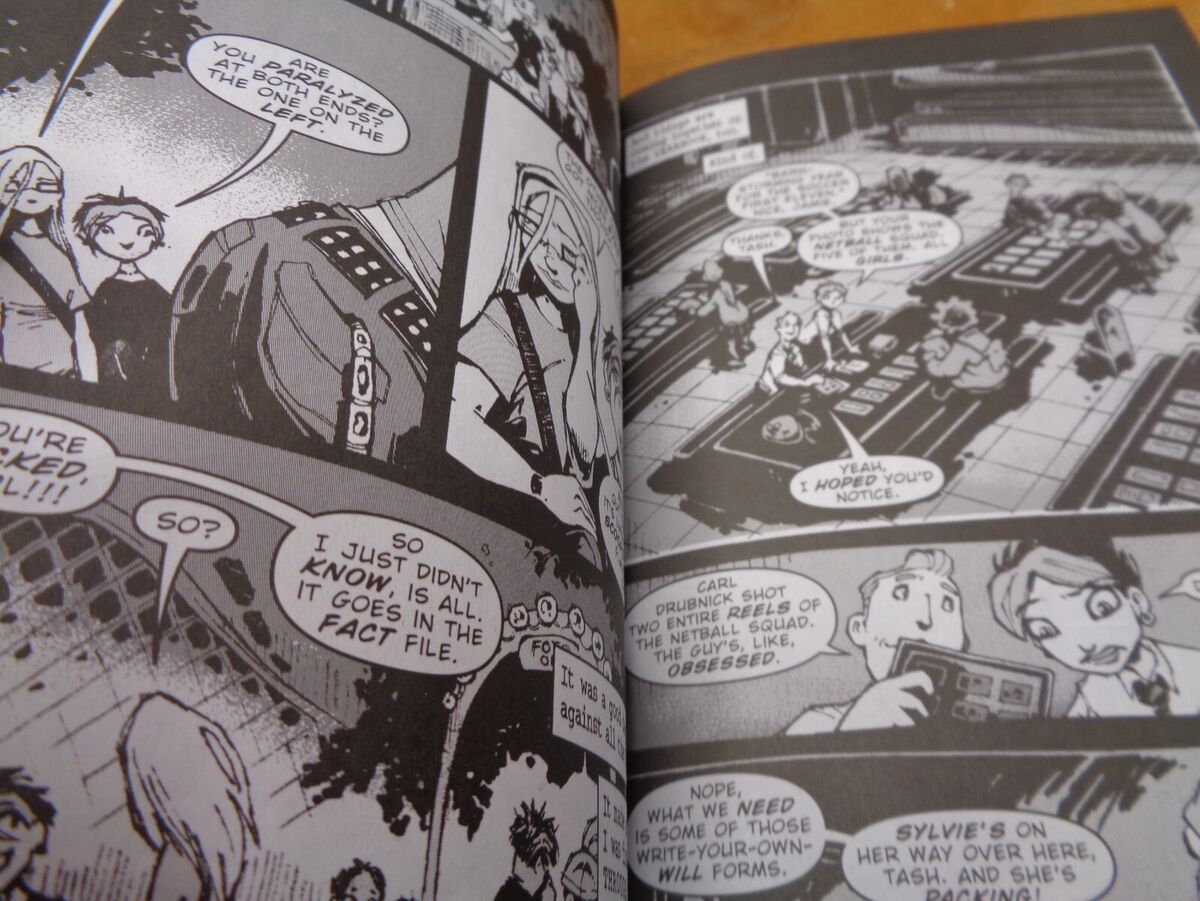The image depicts an open black-and-white comic book, laid out on a medium-toned wooden table. The comic book contains two slightly curved pages with various panels framed by thick black borders. The left page appears to show a school setting, perhaps a cafeteria, where multiple teenagers are engaged in conversation. In the top panel, two girls—one with short blonde hair and another with long blonde hair and square-framed glasses—are watching a person bent over. One girl says, "Are you paralyzed at both ends?" Further dialogue on this page includes snippets like “So, I just didn’t know is all; it goes in the fact file.” 

The right page features varied scenes, with one panel showing a casino where people are playing cards at tables. Among the text, one character comments, "Karl Drebnik shot two entire reels of the netball squad; the guy's like obsessed," while another bubble reads, "Nope, what we need is some of those write-your-own-will forms. Sylvie's on her way over here, Tash, and she's packing." Parts of the dialogue are challenging to read due to the page being slightly out of focus. Overall, the comic book captures typical mid-century comic style and teenage interactions, with elements of humor and casual conversation.